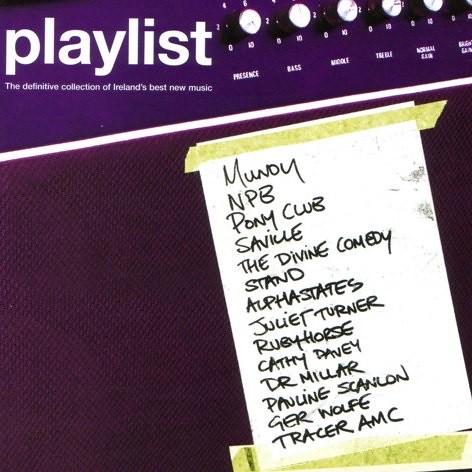The image is a square-format color photograph. At the top left, the word "playlist" appears in lowercase white letters, followed beneath by the smaller text "the definitive collection of Ireland's best new music." The upper background features a purple hue that transitions into a black control panel with visible knobs labeled "Presence," "Bass," "Middle," and "Treble," each numbered from 0 to 10. Below this panel, a white line separates it from a darker purple background. A piece of white paper, attached with yellow tape at the top and bottom, is prominently displayed on this background and contains a handwritten list of names in black letters. The names listed are: Monday, NPB, Pony Club, Saville, The Divine Comedy, Stand, Alpha States, Juliet Turner, Ruby Horse, Kathy Davey, Dr. Millar, Pauline Scanlon, Durer-Wolfe, and Tracer AMC. The overall style of the image is photographic realism.